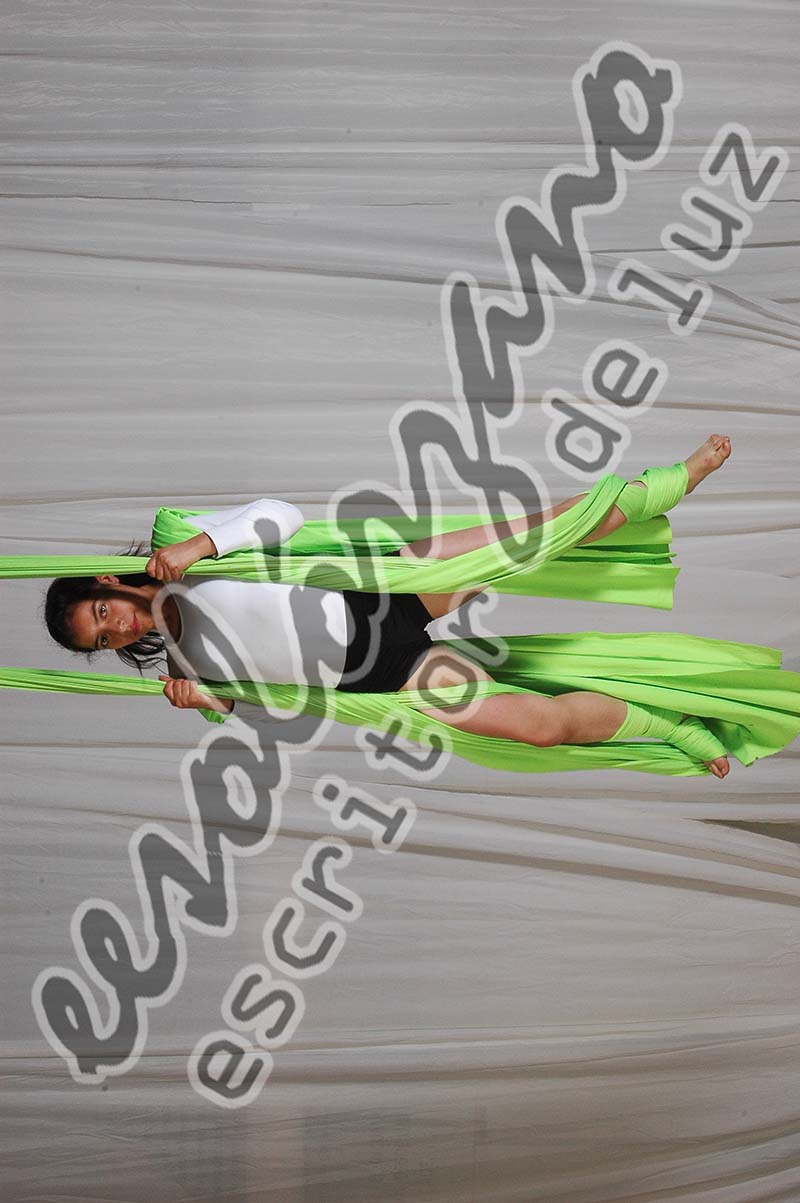In this detailed photograph, a woman with long, dark black hair is gracefully suspended from coils of vibrant, light green fabric, reminiscent of Cirque du Soleil acrobatic displays. The fabric is carefully wrapped around her foot and body, ensuring her balance as she performs a mid-air dance. She is dressed in a white, long-sleeved t-shirt and black shorts, showcasing a striking contrast against the green fabric and the grayish backdrop. Her figure is positioned horizontally across the image, with her head to the left and feet to the right, giving the impression that she is laying down while hanging in the air. The backdrop also includes white fabric, adding layers to the scene. 

Text in a different language, written in a script, spans diagonally across the image, with one of the legible phrases being "Escritor Deluxe." The remaining wording, outlined in white, is difficult to decipher but seems to be part of an advertisement, potentially digitally created. The overall composition, with its blend of dynamic human form, vibrant colors, and mysterious text, exudes an artistic and gymnastic allure.